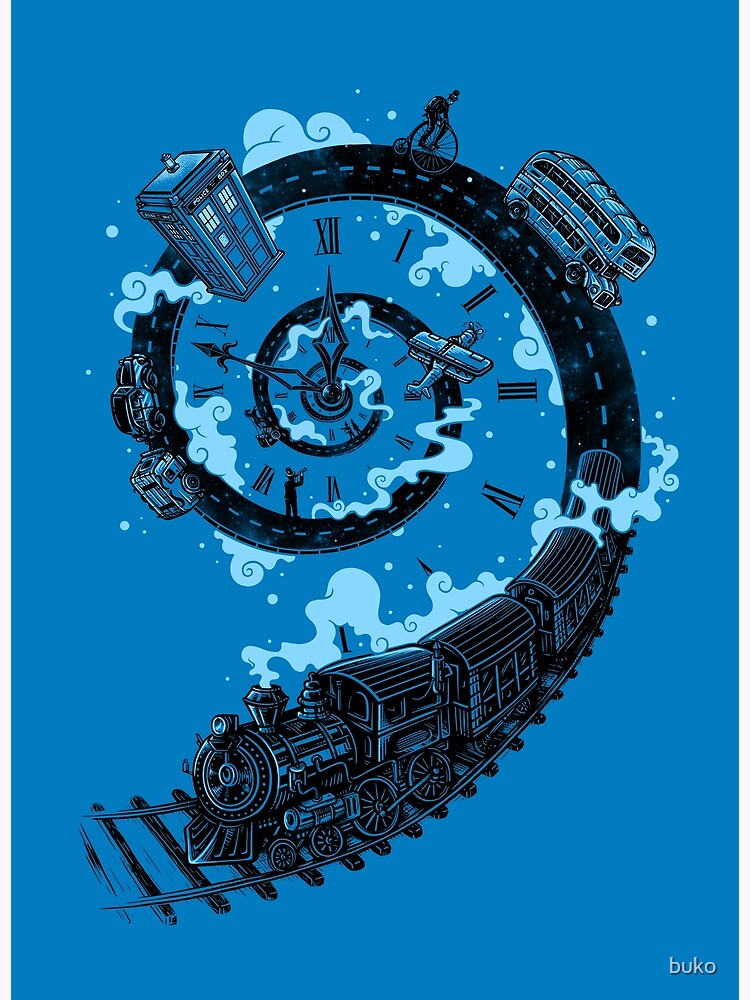Set against a dark blue, artistically rendered digital background, this captivating image showcases a surreal clock composed of a spiraling railroad track that transitions into a road. The spiral originates from the bottom left corner, moving inward and upward, narrowing as it reaches the center where the clock hands are located—one small and wide, pointing upwards, and the other longer and slender, pointing to the left. Adorning the spiral are Roman numerals marking the hours.

From the left, a large, cartoonish black steam engine with three additional cabs makes its way along the train tracks until they morph into a black road marked with red or blue dots. The top right corner of the image features a double-decker bus followed by a man on a unicycle. A blue phone booth, reminiscent of the TARDIS from Doctor Who, is placed nearby. Further along the spiral, various modes of transportation appear in sequence, including a horse and buggy, a car towing a camper, and an airplane flying overhead. Additional details include more cars and a man standing on the road. The composition is encircled by light-colored blue smoke or clouds that add to the whimsy of the scene.

In the bottom right corner, "Buko" is inscribed in white lettering, adding a final artistic touch to this imaginative journey through different eras and modes of travel, all seamlessly integrated into a functional clock.